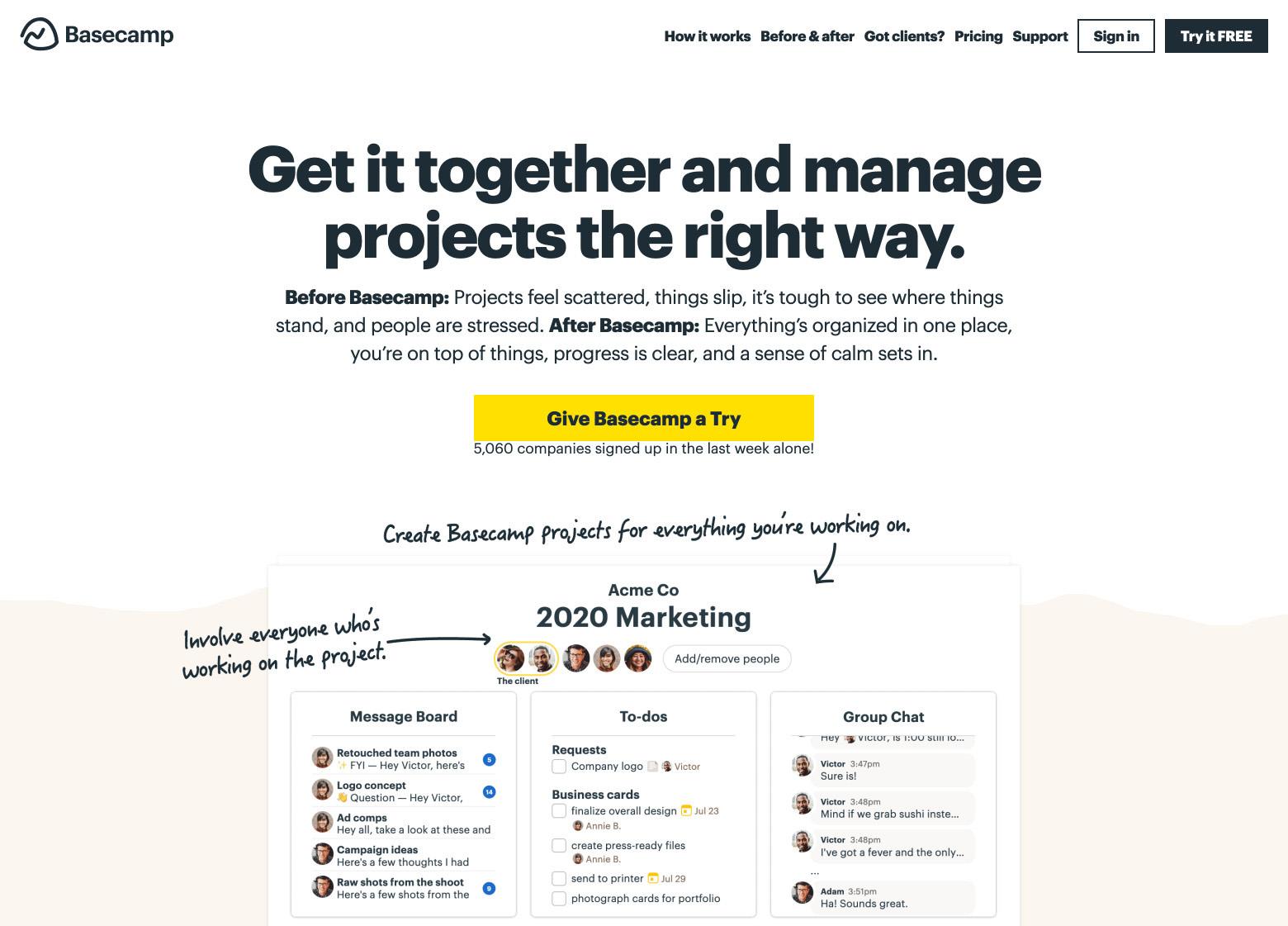In the upper portion of the screen, set against a white background, a small mountain icon is positioned in the top left corner beside the word "Basecamp." To the right, a navigation menu includes links titled "How it Works," "Before and After," "Got Clients?" (with a question mark), "Pricing," and "Support." Below this, there are two buttons: one white with black font labeled "Sign In," and the other black with white font labeled "Try it Free."

The main header reads, "Get it together and manage projects the right way." Below it, a brief narrative explains the benefits of using Basecamp: "Before Basecamp, projects feel scattered, things slip. It's tough to see where things stand and people are stressed. After Basecamp, everything's organized in one place and you're on top of things. Progress is clear and a sense of calm sets in." Positioned below this text is a yellow button that encourages users to "Give Basecamp a try," highlighting that "5,060 companies signed up in the last week alone."

Further down, a section instructs users to "Create Basecamp projects for everything you're working on" with an arrow pointing downward. Adjacent to this is another prompt, "Involve everyone who's working on the project," with an arrow pointing to the right. Below these instructions, an example project titled "Acme Company 2020 Marketing" is displayed, featuring five profile images. The option to "Add/Remove People" is visible, with two highlighted profiles labeled "The Client." The interface also showcases a message board, a to-do list, and a group chat filled with various information, illustrating Basecamp's functionality.